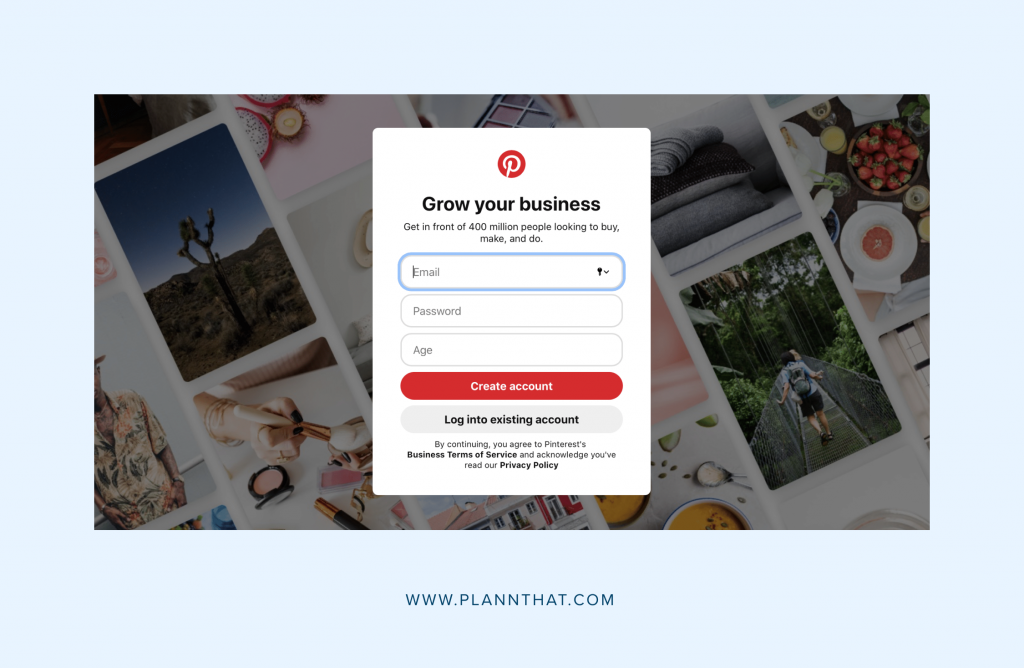The image features a blue background with a central square representing a pop-up window for Pinterest account creation or login. Surrounding this window are small, vividly detailed photographs depicting various items and activities: a cactus, a woman applying makeup, a plate of food, a woman walking across a bridge, a woman wearing a dress, a collection of pillows, and another plate of food with strawberries. At the bottom of the blue background, the URL www.planthat.com is displayed, adding a web address element to the composition.